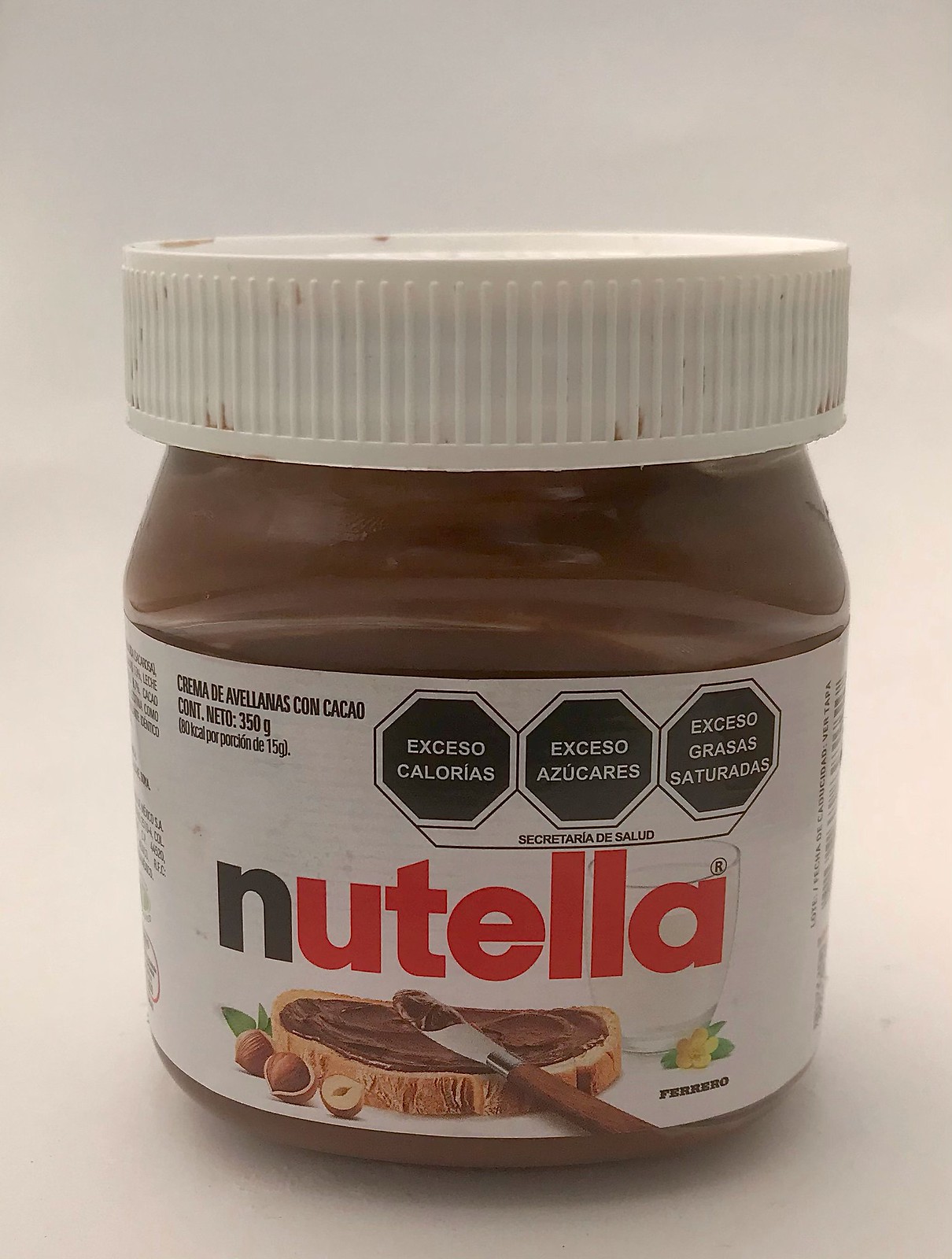This is a professionally taken close-up photo of an unopened Nutella jar with a white lid, set against a beige backdrop. The jar appears full, revealing the brown Nutella inside. The Nutella logo, written in red and black on a white label, is central to the image. Above the logo are several descriptive boxes in black with white text, with phrases like "Exceso Calorias" and "Exceso Azucares," suggesting the label is in Spanish or another non-English language. Below the logo, there is an image of a piece of bread with Nutella being spread on it by a knife, surrounded by open nuts on the left and a glass with a small yellow flower to the right. The lid shows some brown flecks, possibly indicating it was touched by Nutella-coated hands. The brand "FERRERO" is displayed beneath the image on the label.